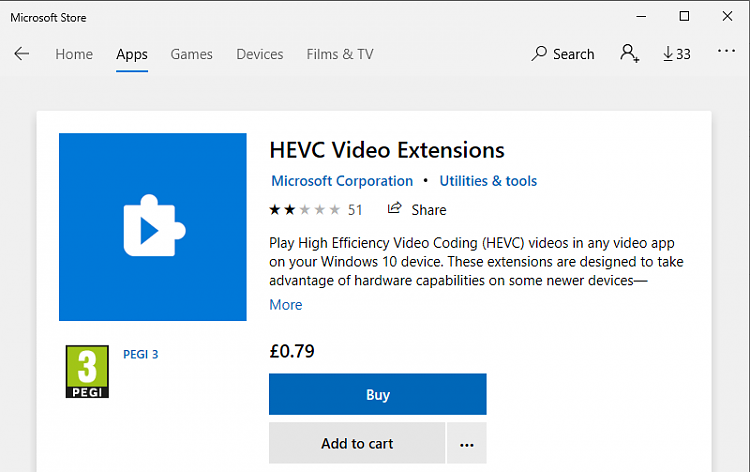The image displays a detailed view of a specific listing on the Microsoft Store interface with various navigational and functional elements. At the top, there are menu tabs labeled "Microsoft Store," "Home," "Apps," "Games," "Devices," "Films," and "TV." To the right of these tabs, there is a search bar accompanied by a magnifying glass icon, a person icon with a plus sign, a downward arrow, the number "33," and an icon with three horizontal dots.

Central to the image is a blue square icon featuring a white puzzle piece with a blue triangle, representing the "HEVC Video Extensions" by Microsoft Corporation. This item is categorized under "Utilities & Tools." A star rating system is depicted, with five stars where two are filled in, and the number "51" indicating the count of ratings.

Below the item description, there is a share icon followed by the text "Share." The main description reads, "Play High Efficiency Video Coding (HEVC) Videos in any video app on your Windows 10 device. These extensions are designed to take advantage of hardware capabilities on some newer devices." Following this, there is a "More" link in blue text.

The price for the extension is listed as "$0.79" or "79 cents," with purchasing options including a blue "Buy" button with white text, and an "Add to cart" button in black text on a gray rectangle. Adjacent to these buttons is a light gray square with three black vertical dots.

Overall, the image provides a comprehensive and user-friendly layout, facilitating easy navigation and understanding of the HEVC Video Extensions listing on the Microsoft Store.